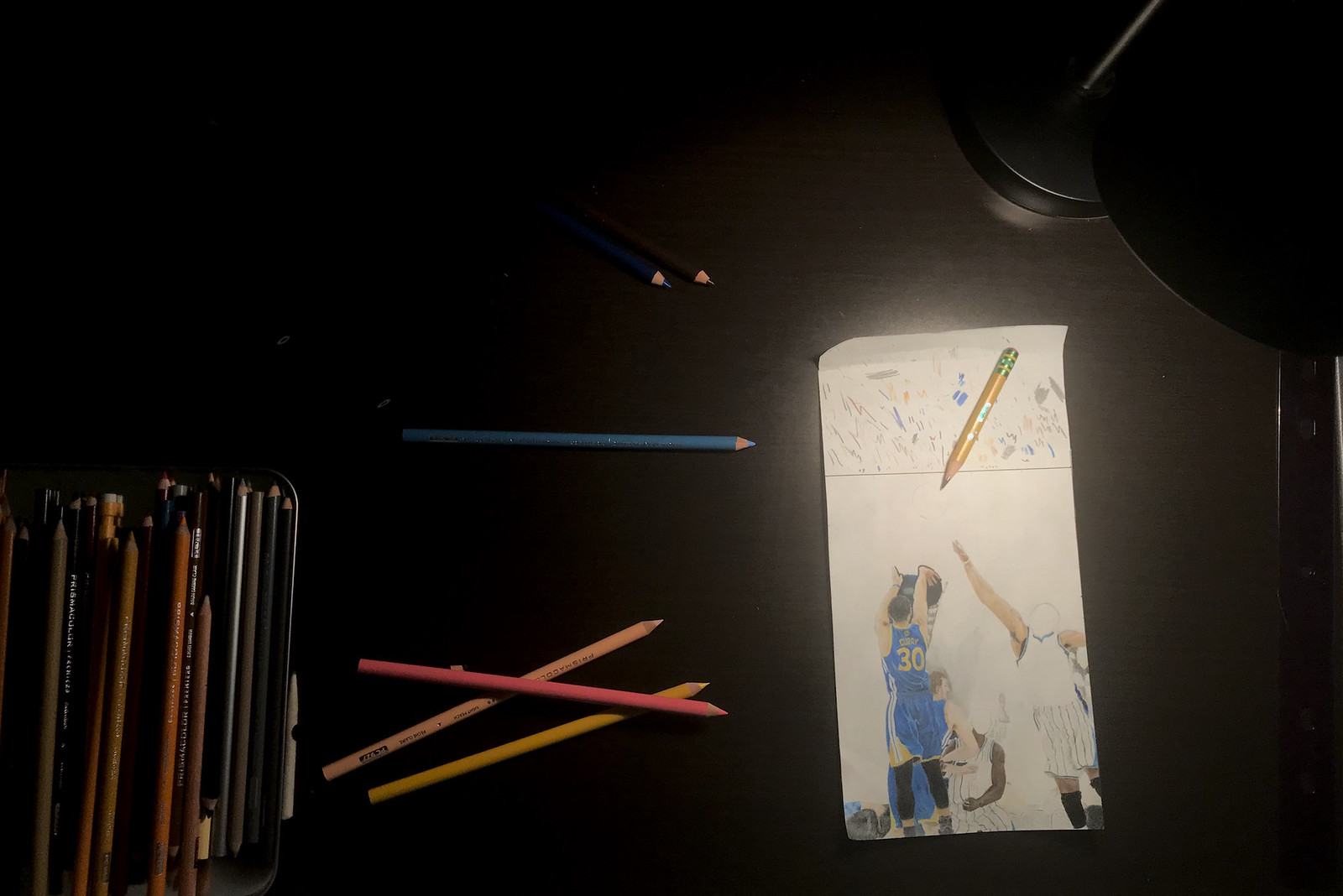This photo captures a detailed and immersive scene on a dark brown wooden desk. Illuminated solely by the light of a black desk lamp, the photo showcases an intricately drawn basketball game on a large white piece of paper. The focused lamp light accentuates a highly realistic sketch of a basketball player—depicted as Steph Curry—wearing a blue and gold number 30 jersey and black leggings, making a jump shot. Another player in a white uniform with black stripes, whose head is unfinished, attempts to block the shot. The drawing also features additional players, one notably a teammate of Curry’s. 

Scattered across the scene, primarily on the left side of the desk, is an array of colored pencils. Four colored pencils lay horizontally near the drawing—a pink pencil atop two shades of yellow and a blue pencil—while numerous others are vertically bunched together in the lower left corner. A much-used, short yellow number two pencil lies across the top of the paper. The paper also bears a small band of test colors at the top edge, suggestive of careful prepping for the artwork. This highly detailed and artistically arranged desk gives a glimpse into a creator’s workspace amid the process of bringing a vivid moment of a basketball game to life.